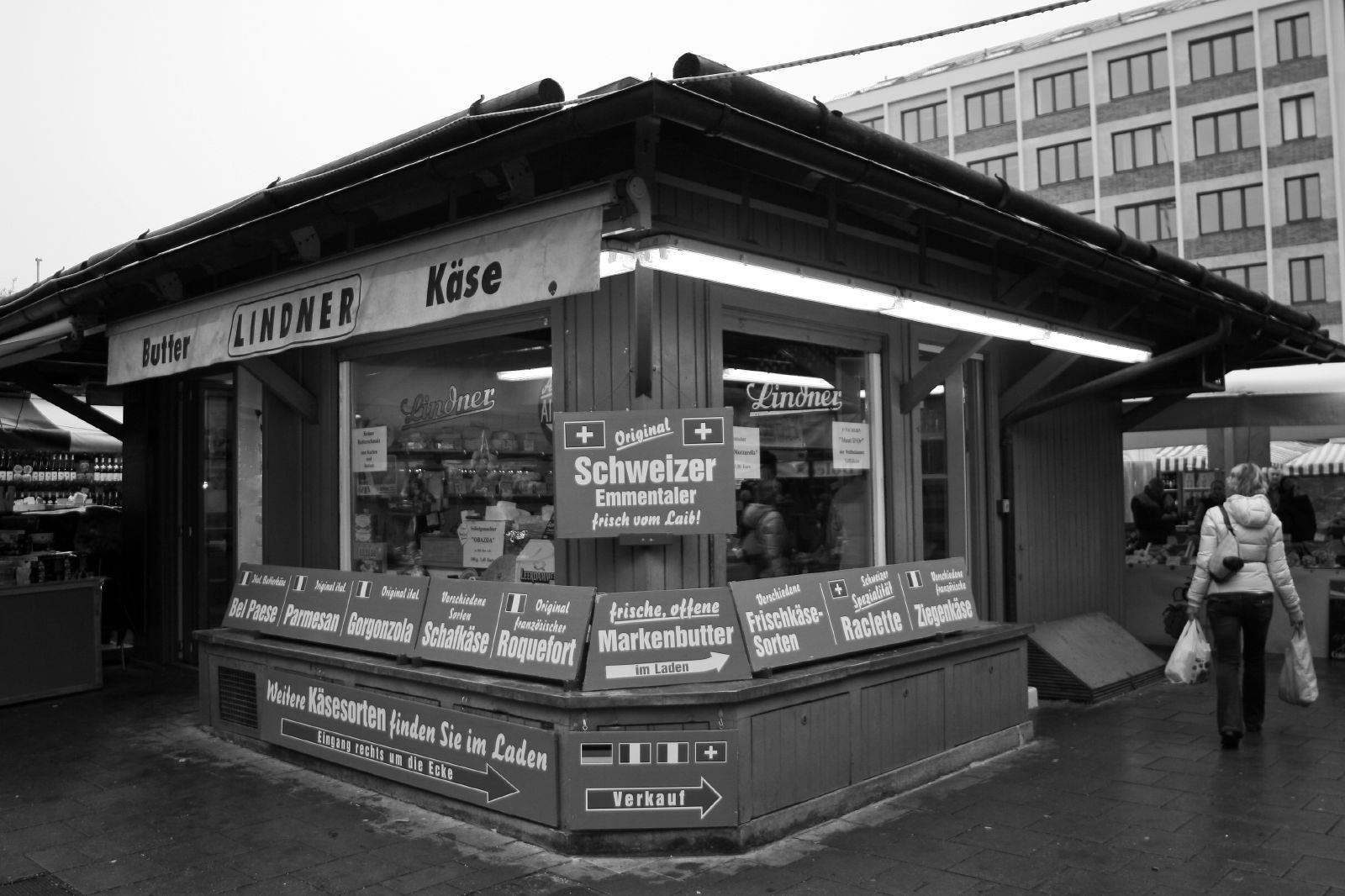The image is a high-resolution black and white photograph of a unique, standalone, triangular-shaped store, designed to look like an old-timey diner. Located at an angled corner, the building, likely in Germany given the umlauts in the signage and the visible German flag, has a distinctly retro appearance. The store displays several signs with German text, including "Schweitzer Emmentator," "Original," and "Lindner Kase." A small overhanging roof tops the structure, with four prominent picture windows allowing glimpses inside, though the details are too distant to discern. The bright lighting around the store highlights various advertisements. To the right, a woman dressed in a white down jacket and dark pants walks along the sidewalk, carrying two white grocery bags and a pocketbook. The scene suggests a 1950s or 60s setting, reinforced by the woman's attire. In the background, there's a multi-story apartment building, adding to the urban atmosphere. The storefront, surrounded by additional buildings, stands out as an inviting spot, perhaps offering cheese, meats, or other foods typical of a mid-century German market.